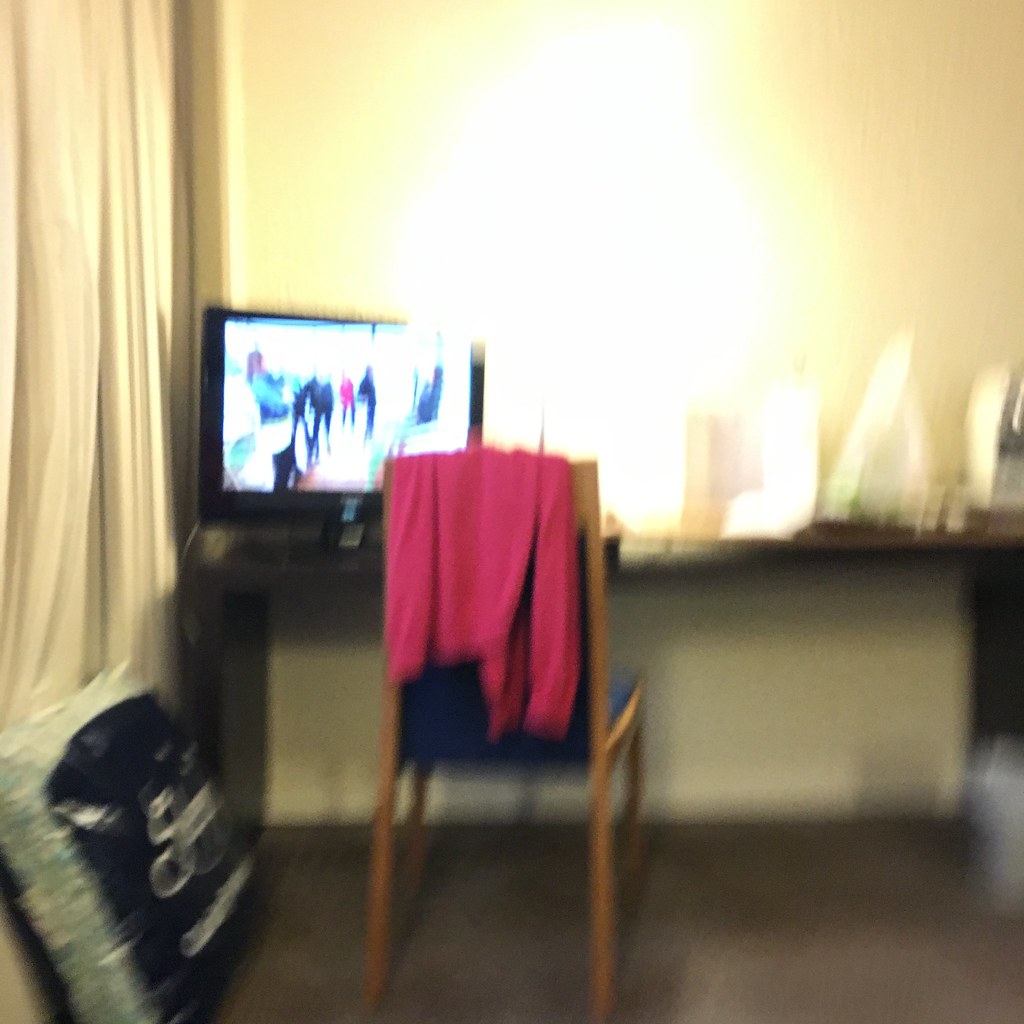This image is a poorly shot and blurry photograph of a room. On the left-hand side, floor-length white curtains cover a window or possibly a doorway. Nearby, there is a large blue and white plastic bag with unreadable white text on it, likely containing bedding or a pillow. The focal point is a long desk, possibly wall-mounted, with a TV or computer monitor displaying indistinct images of people. In front of the desk is a wooden chair with blue cushions, draped with a pink sweater. The desk holds various indistinct, white-blurred objects. A glaring, golden light source illuminates the center wall above the TV. The far right corner of the image shows a white and blurred object on the ground underneath the desk. The room has white walls and a carpeted floor.